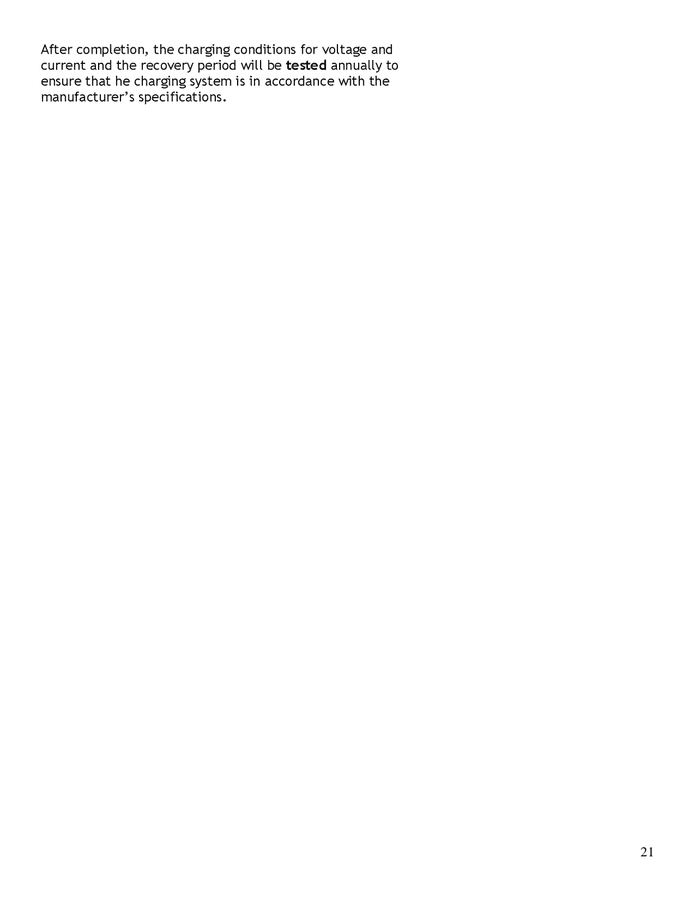This image displays a text paragraph in black font on a white background. The paragraph comprises four lines and contains a comma, a period, and an apostrophe. The first word of the paragraph is "After," which begins with a capital 'A'. The sentence reads: "After completion, the charging conditions for voltage and current and the recovery period will be tested annually to ensure that the heat charging system is in accordance with the manufacturer's specifications." Additionally, a black number '21' is positioned in the lower right-hand corner of the image.